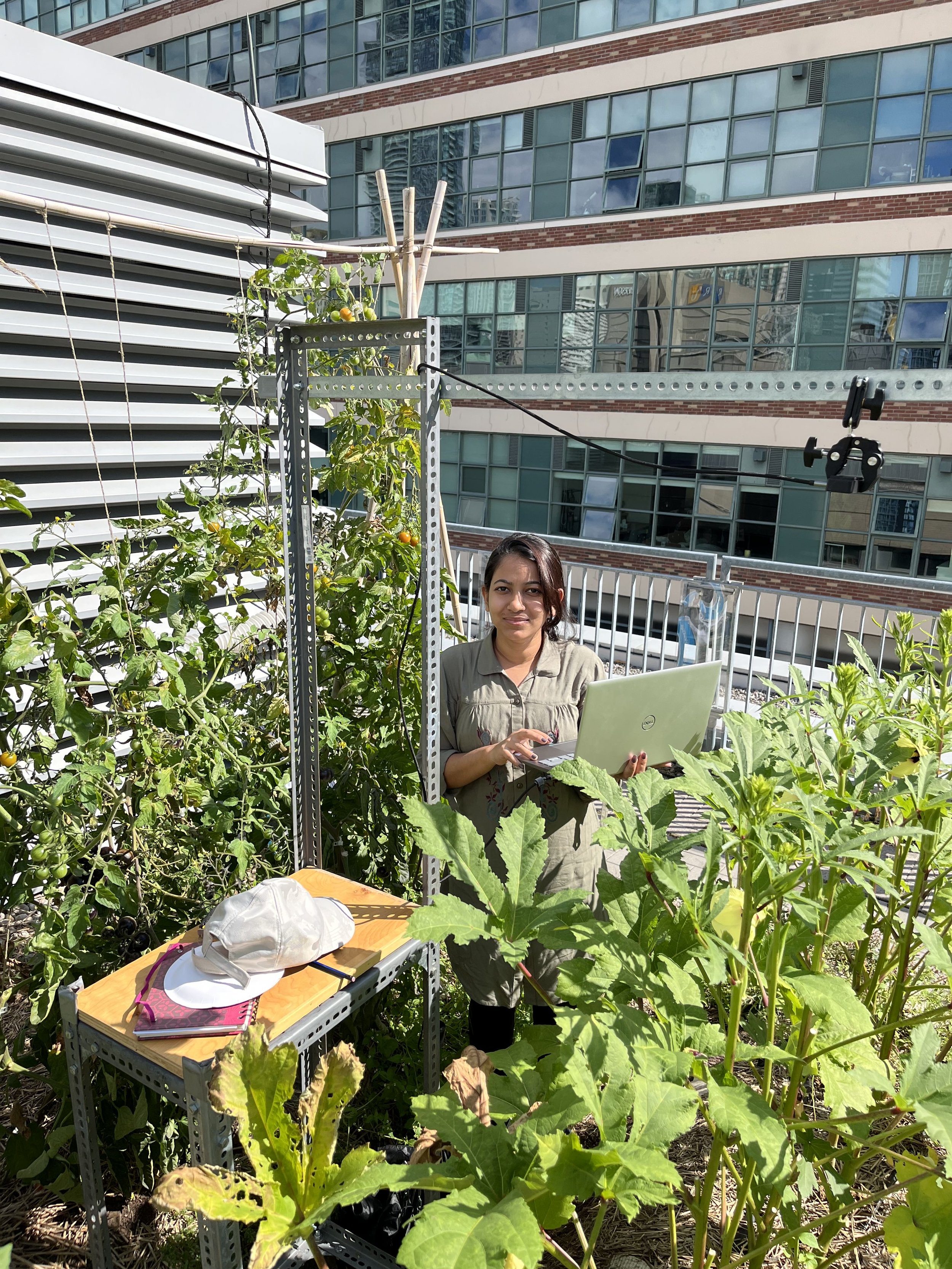This detailed photograph captures a woman standing amidst a lush rooftop garden, perched atop a high-rise building. She is holding an open laptop, secured with her left hand while her right hand rests on the top of the keyboard. The surrounding garden boasts a variety of tall, green plants that reach up to her shoulders, epitomizing a thriving urban oasis. In the background, the scene is framed by towering buildings, with one notably higher than the rest and a commercial AC unit seen to her left. She has short, dark hair, and wears a gray shirt, her complexion marked by a healthy tan. Beside her stands a small, wooden table set on a metal stand, upon which a white baseball cap and a notebook are placed. The scene is bathed in daylight, providing a clear, vibrant view of the garden's greenery. The woman's presence, coupled with the laptop and natural surroundings, suggests she might be a researcher dedicated to studying urban horticulture.